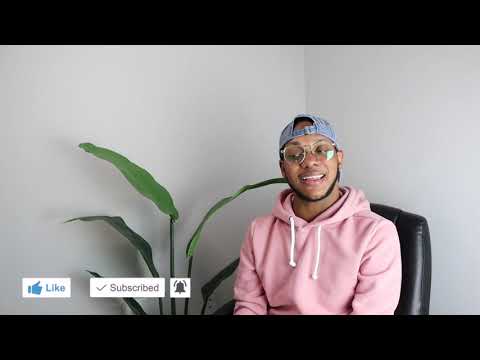The image is a screenshot from a social media video, featuring a man sitting in a black leather office chair. The man appears to be of African American or Latino descent, with a dark complexion. He is wearing prescription glasses and a backwards denim baseball cap. His facial hair includes black stubble and a light mustache that frames his face, which is mid-sentence with his mouth open. He is dressed in a light pink hooded sweatshirt with white drawstrings hanging down. 

Behind him is an off-white or light gray wall, and to his right (the viewer's left), there is a green plant with several large, floppy leaves, though the pot is not visible. In the lower left corner of the image, there is a white rectangle containing three interactive icons: a blue thumbs-up with the word "like," a checkmark with the word "subscribed," and a black bell icon. The overall composition suggests that the man is a social media influencer or content creator.